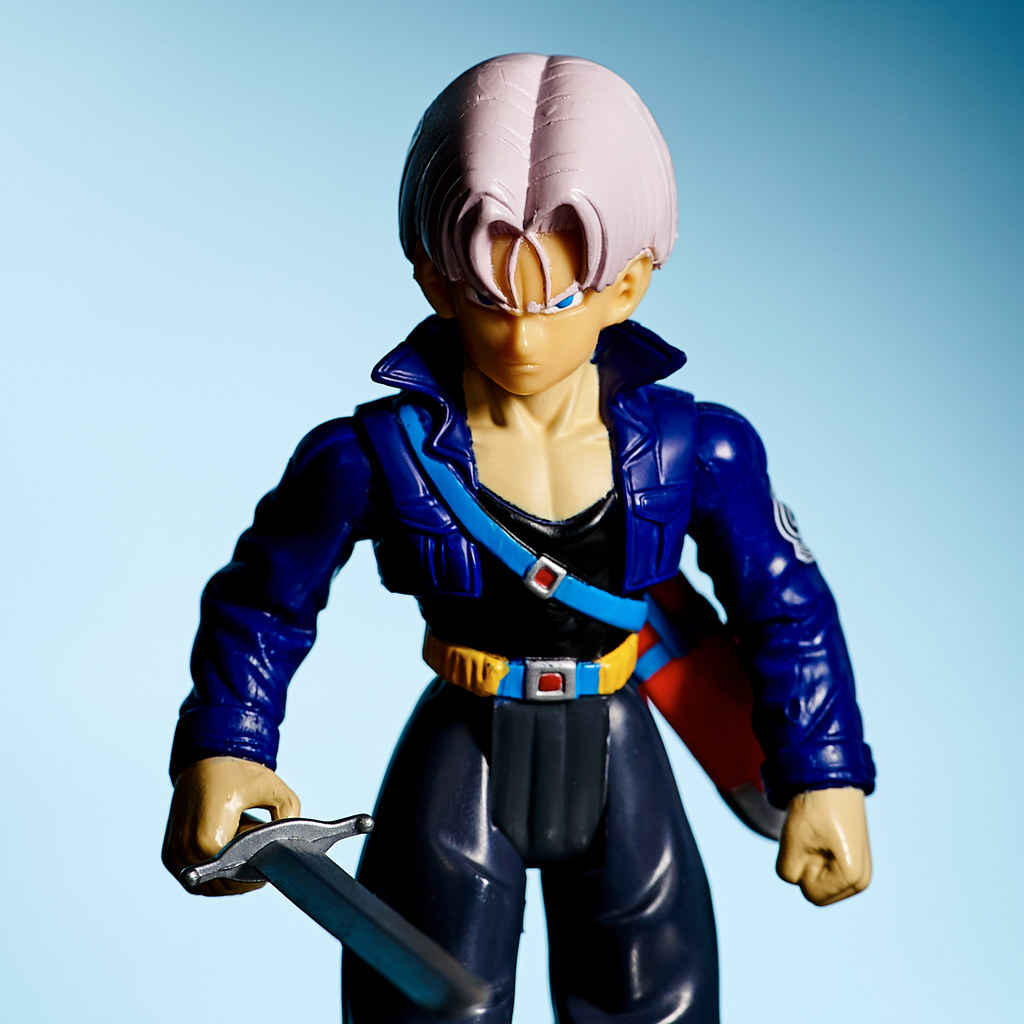This color photograph features a highly detailed plastic action figure of the Dragon Ball Z character, Trunks, set against a pale blue background. The figure depicts Trunks in a dynamic stance, with his right hand firmly gripping a sword, while the scabbard is strapped across his chest in a style reminiscent of Rambo. Trunks is dressed in a blue jacket over a black tank top, accompanied by black pants and a distinctive yellow, blue, silver, and red belt. His finely crafted blonde hair, parted severely down the center, appears almost white or gray in some lights, and contrasts with his stern blue eyes, which are slanted downward, adding to his serious expression. Painted with intricate attention to detail, the figure shows some minor paint defects, and is illuminated with two-point lighting to highlight its features.